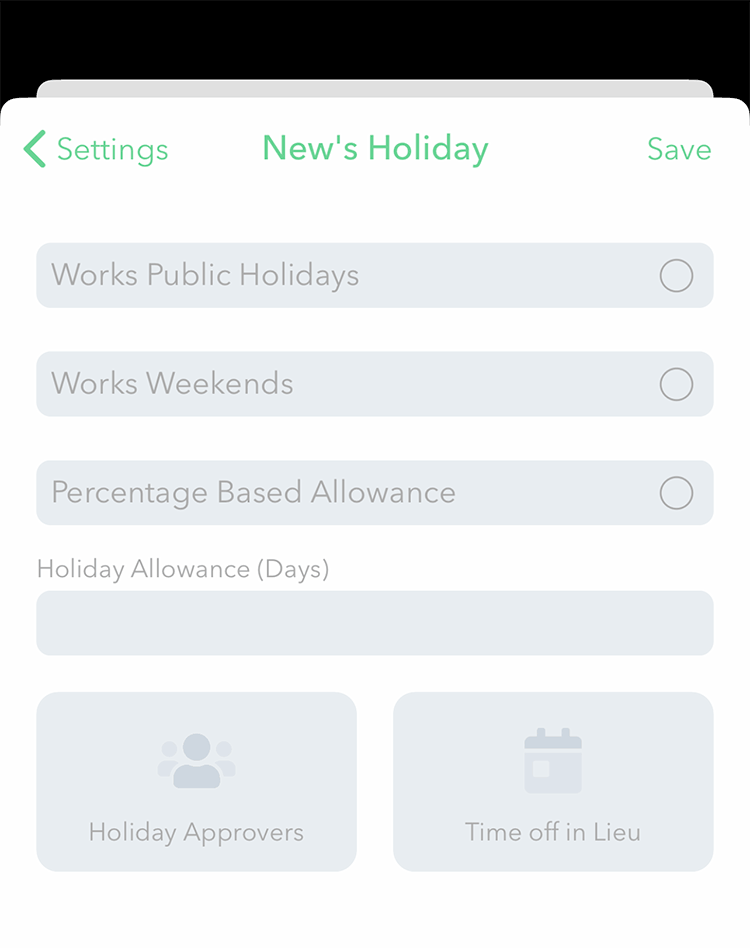In the image, there is a user interface with various icons and text elements set against a predominantly gray background. At the top, there's a gray bar featuring a left arrow, followed by icons for settings and a 'Holiday' label centered prominently. To the right, the bar includes options such as 'Works', 'Public Holiday', and 'Weekends', all indicated with gray text.

Below this bar, there's an oval labeled 'Percentage-Based Allowance', emphasizing 'Holiday Allowance'. Adjacent to this is a square labeled 'Holiday Approvals', also gray, and an icon depicting a person. The interface appears to include an interactive calendar alongside elements linked to 'Time Off in Lieu' and ticket booking, possibly for homes or vacation rentals.

The background is mostly white, contrasting with the gray elements. The central theme revolves around holiday settings, approvals, and allowances, with consistent gray color usage throughout various interactive components.